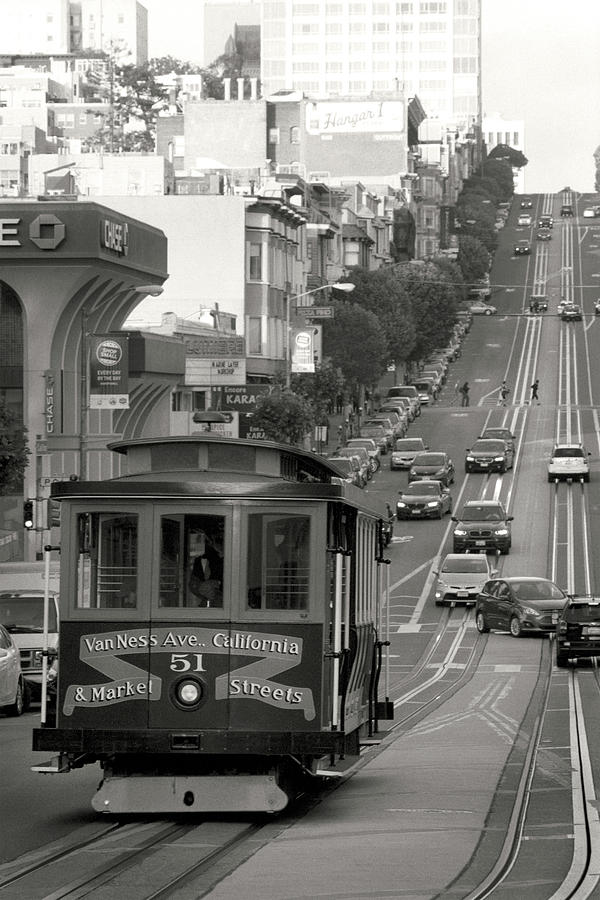This detailed black-and-white photograph captures a quintessential San Francisco scene, bustling with activity. Dominating the foreground is a classic San Francisco cable car numbered 51, prominently displaying the routes "Van Ness Avenue," "California," and "Market Streets." The cable car, iconic in its presence, seems poised at the base of a steep hill, characteristic of San Francisco's hilly topography. Adjacent to the cable car, a Chase Bank building stands on the left, accompanied by several other commercial establishments stretching into the distance. The street is alive with numerous cars navigating the busy traffic, both ascending and descending the hill. Trees planted along the sidewalks add an organic touch amidst the urban landscape, while streetlights and advertisements further accentuate the city's vibrant scene. In the far background, pedestrians cross the road, contributing to the overall sense of a bustling, modern city despite the photo's monochromatic palette.